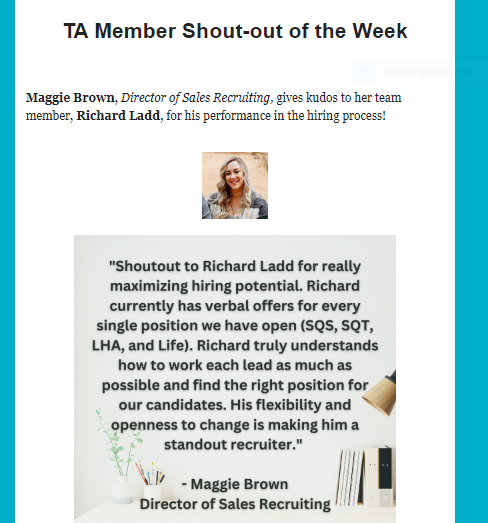The image is a detailed flyer recognizing the "TA Member Shout Out of the Week." It features a vibrant, centrally-placed picture of Maggie Brown, the Director of Sales Recruiting, smiling and wearing a blue jacket with a silver necklace. Flanking the white background are vertical blue borders on the left and right sides, framing the content. The top of the flyer prominently displays black text that reads "TA Member Shout Out of the Week." Below Maggie’s picture, a grey box contains more black text, giving special kudos to her team member, Richard Ladd, for his outstanding performance in the hiring process. The text highlights Richard’s significant achievement of securing verbal offers for every open position within the company, including SQS, SQT, LHA, and LIFE. Maggie praises his ability to maximize hiring potential, flexibility, and adaptability, which make him a standout recruiter. The flyer is further adorned with a few decorative elements such as a lamp, books, a plant, and a container of pens and pencils, creating an inviting and professional appearance.